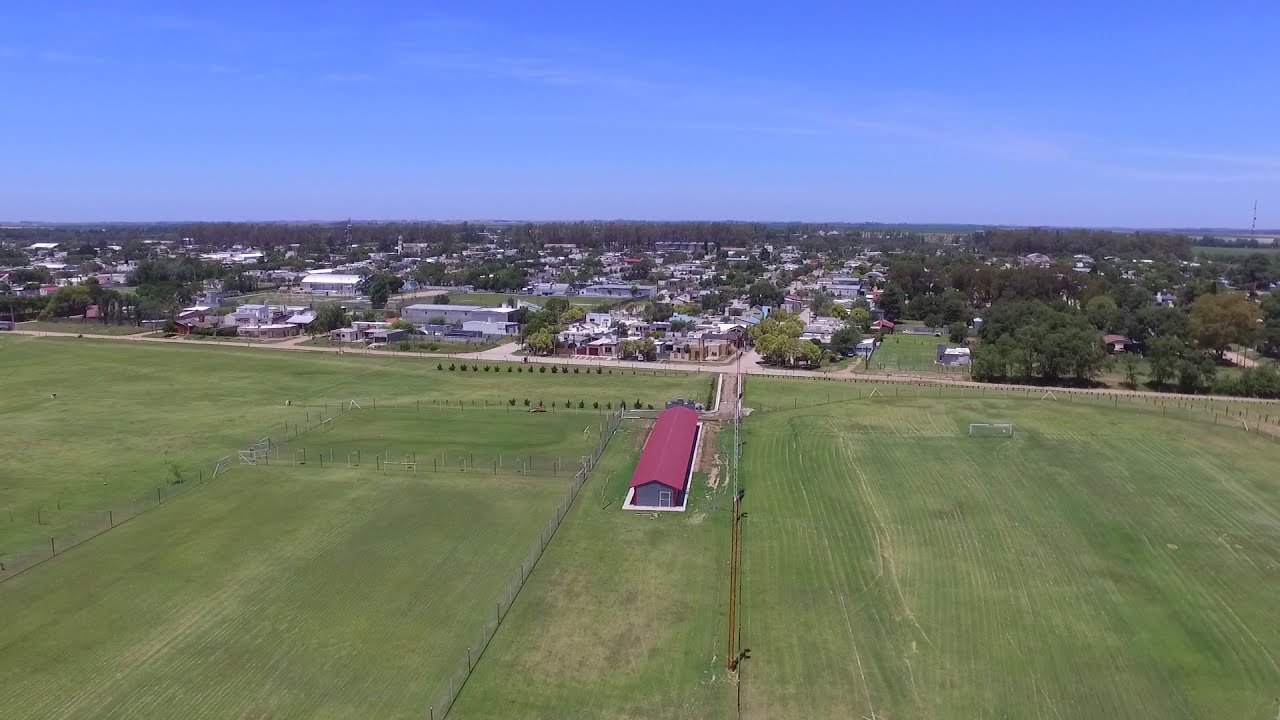The image is a stunning aerial color photograph in landscape orientation, depicting a sprawling grassy field that occupies the foreground and extends the entire width of the image. Central to the scene is a long, red-roofed barn positioned on what appears to be a white platform. A wooden fence meanders through the field, adding structure to the vast expanse of well-manicured grass. Beyond the field and separated by a road, a small town with clusters of white and blue houses sprawls across a valley, interspersed with commercial buildings and verdant trees. The vivid blue sky overhead enhances the vibrant green of the pasture, contributing to the picturesque quality of this drone-captured scene.